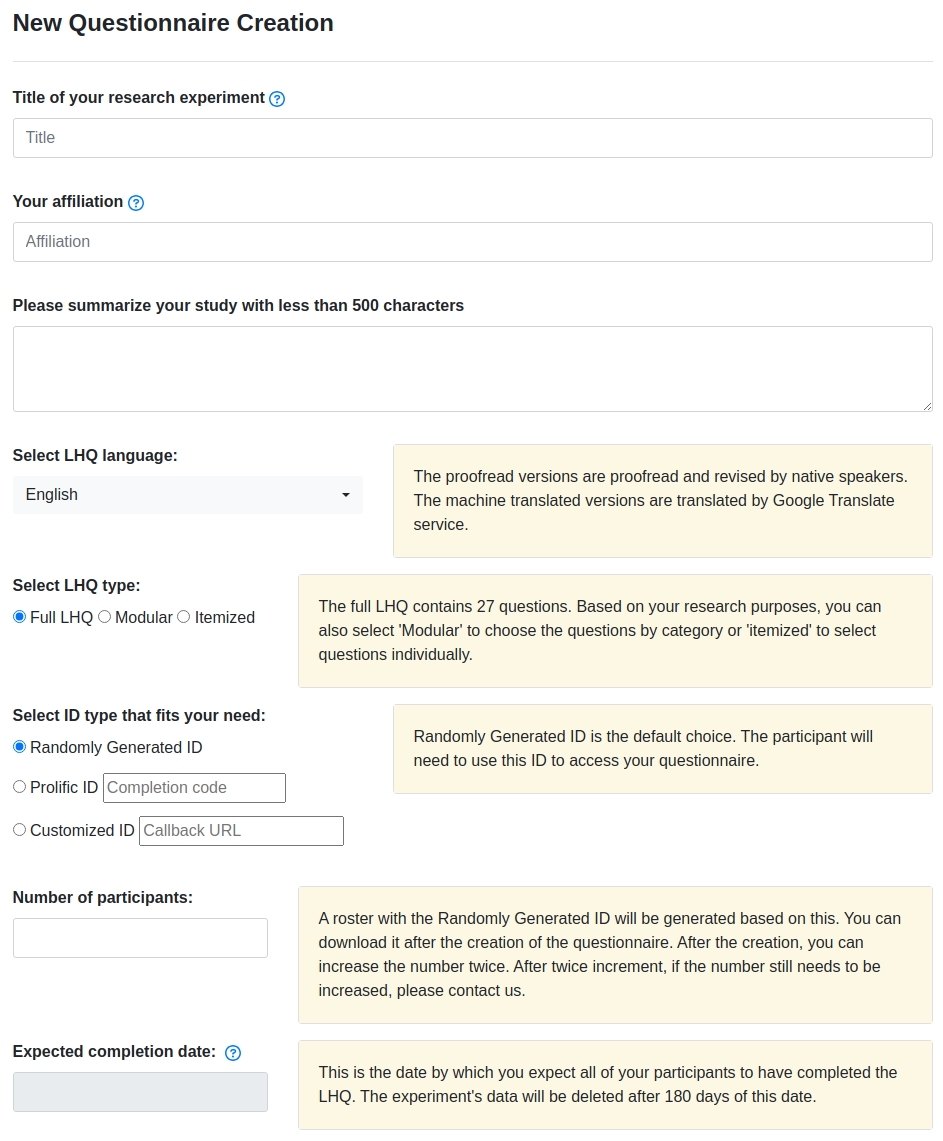This image is a screenshot from a website illustrating the interface for creating a new questionnaire. At the top, there is a header titled "New Questionnaire Creation." Below this header, various input fields are displayed. The first input field is for the "Title of Your Research Experiment," accompanied by a blue question mark icon that provides additional guidance when clicked.

Following this, there's an "Affiliation" field, also with a blue question mark icon for clarification. Beneath these fields is a larger text box labeled "Please summarize your study with less than 500 characters." 

Next, there is a dropdown menu to select the "Language Preference," adjacent to a light yellow text box that explains: "The proofread versions are revised by native speakers, whereas the machine-translated versions are done by Google Translate."

Continuing downward, the user can choose the "LHQ Type," with the option "Full LHQ" currently selected. Other available options include "Modular" and "Itemized."

Following the LHQ selection, users can select the "ID Type" that meets their needs, with "Randomly Generated ID" currently chosen. Additional options include "Prolific ID" and "Customized ID."

Further down, there is a text box titled "Number of Participants" for entering the desired number of study participants. The final item on the interface is "Expected Completion Date," which also features a blue question mark for further assistance.